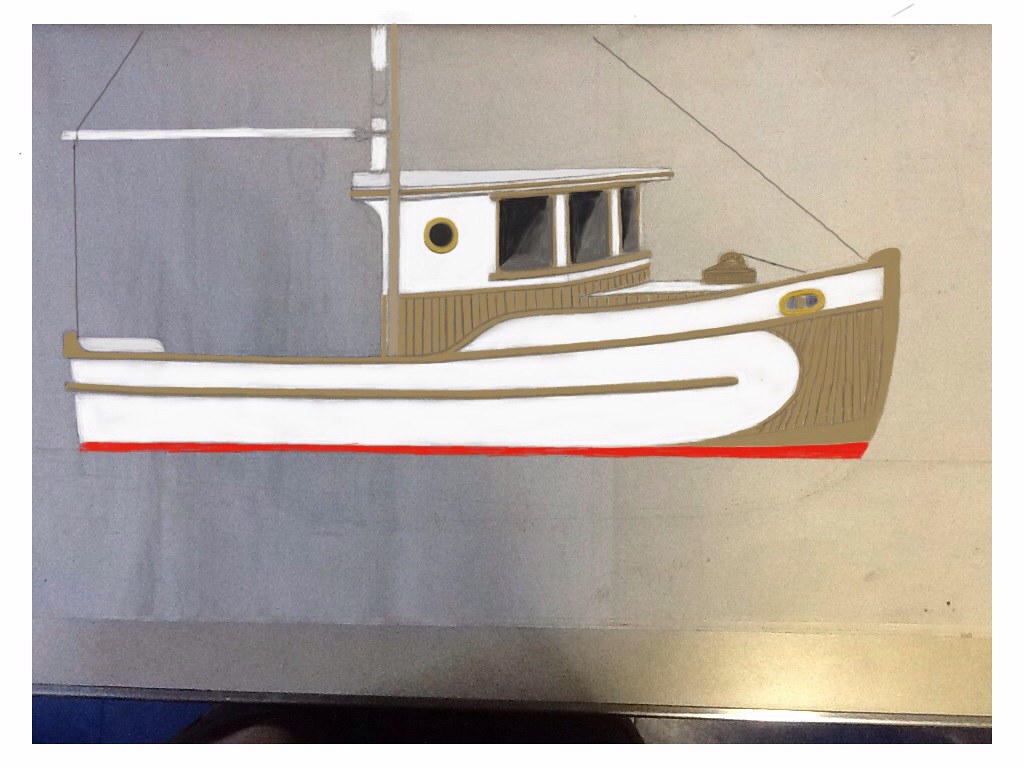This image features a detailed, artistic representation of a small wooden boat, seemingly part of a framed piece of artwork. The boat, which is depicted with a front (bow) facing the right and a rear (stern) on the left, features a white and brown pattern along its sides and red coloring on its bottom. Prominently, the boat showcases three square windows at the front and a circular window beside them. Additionally, ropes can be seen extending from the boat. The entire artwork appears to be set against a white background, with a line of black near the bottom, and a dark blue element in the bottom left corner. The image itself is square-shaped, and the boat has an "S" logo emblazoned across it, suggesting a detailed hand-drawn or digitally-altered effect.